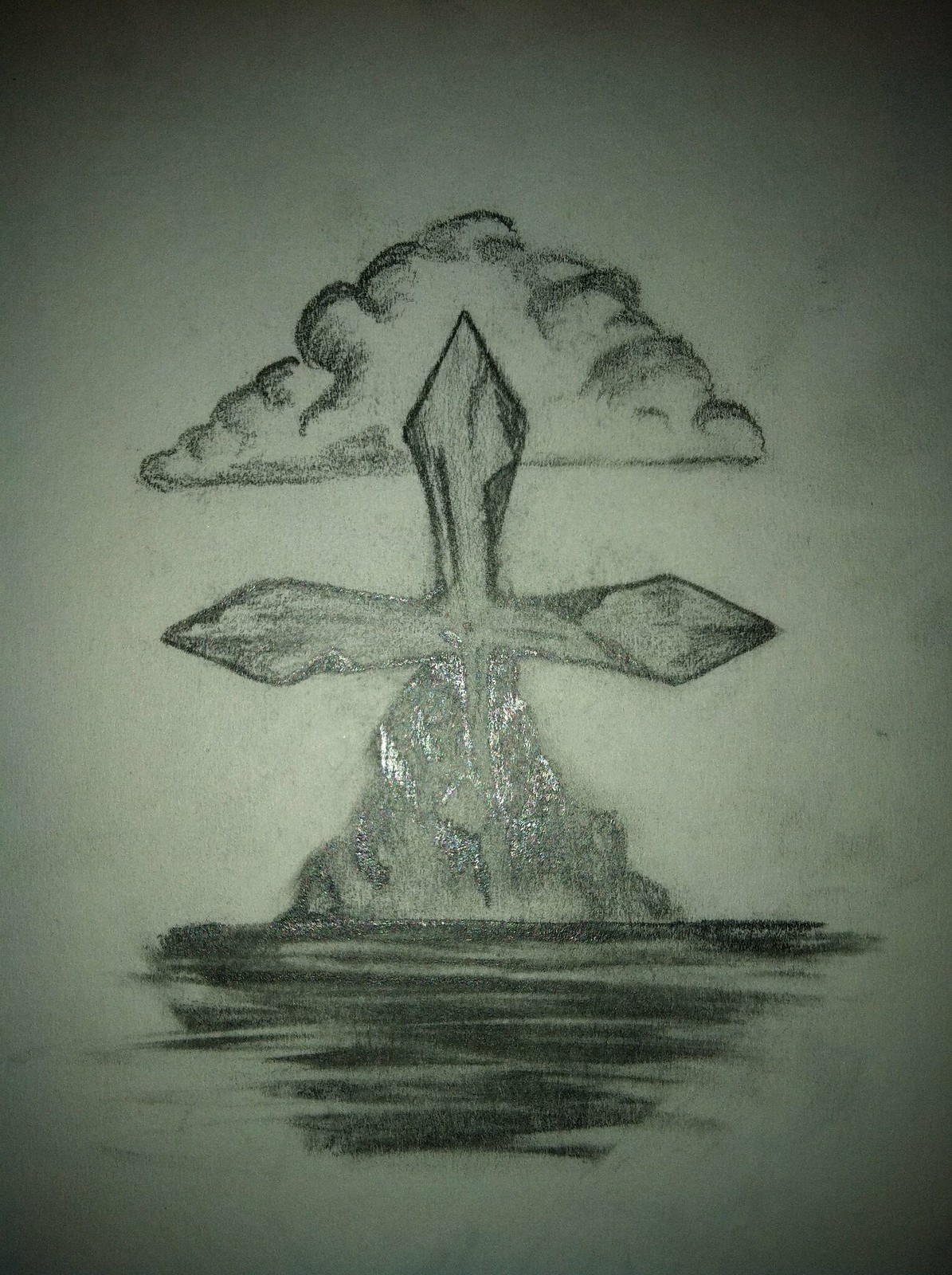The image is a colored photograph of a white sketch pad featuring a detailed pencil drawing. The composition is vertically oriented, and the focal point of the drawing is a thick, bold cross that protrudes from a mound resembling a small mountain or perhaps a volcanic structure. This cross is distinctive due to its arrowhead-shaped endpoints on the horizontal and top portions.

Directly behind the cross, a single cloud is drawn with a flat base and a poofy top. The mound from which the cross emerges has a somewhat rectangular and rough, bumpy texture, suggesting a formation of rocks. Below this mound, the ground is shaded with dark pencil sketches to create a shadow effect, with areas especially darkened in the upper right, lower right, and all four corners of the page, thereby drawing more attention to the central cross and mound.

The entire scene is devoid of any text or other written elements, and the corners of the image are shaded in gray and black, further emphasizing the central elements of the cross and mound. Additionally, there are some gray and brown smudges, particularly on the right-hand side of the paper, adding a touch of texture and depth to the background.